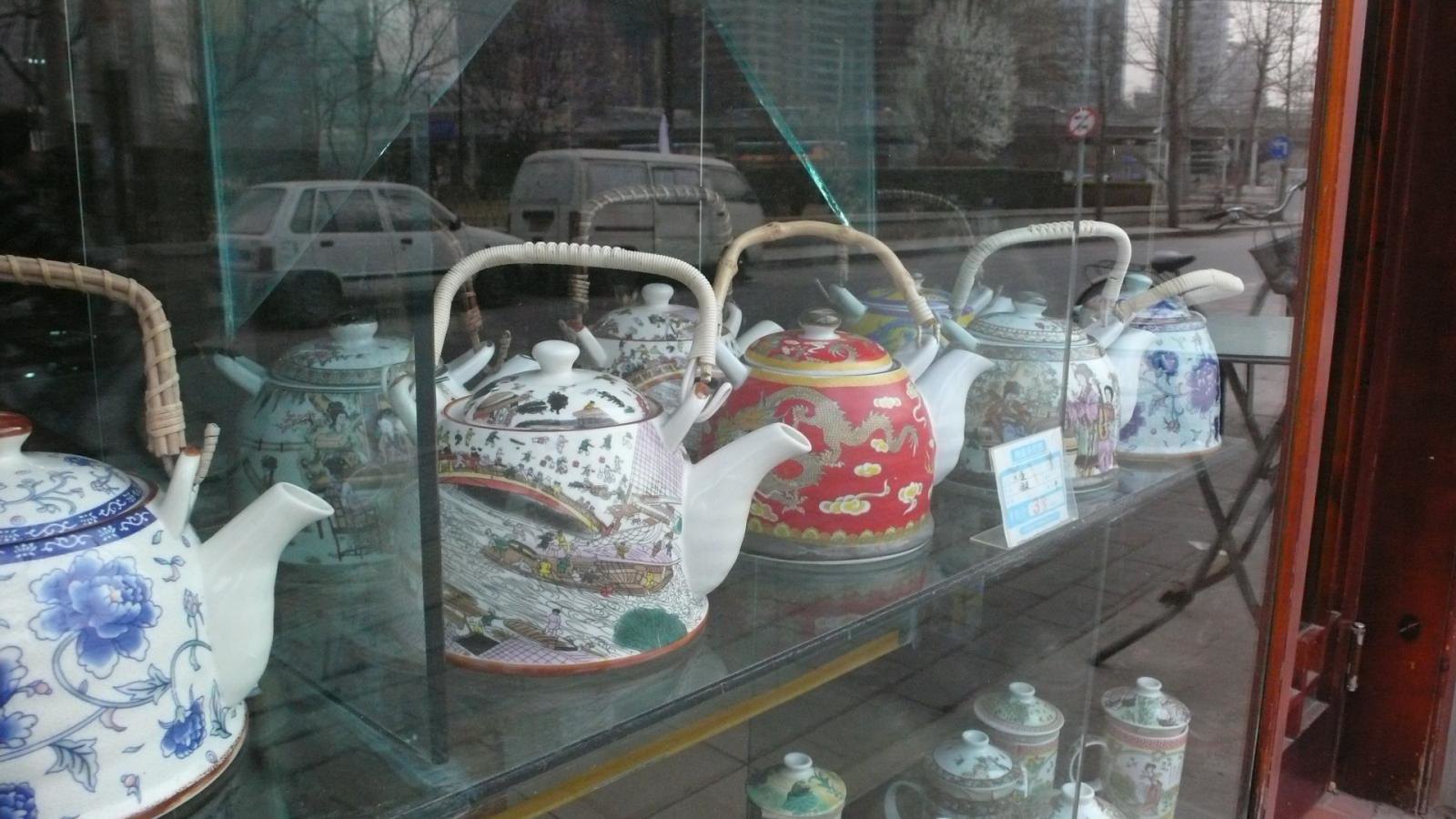This is a color photograph taken from the sidewalk, peering through a storefront’s plate glass window at an artfully arranged display of porcelain teapots. The teapots, which all feature classic Asian designs, are meticulously placed on clear glass shelves within the store. 

Prominently, on the left side of the photo, a white teapot with a blue floral design is housed in a separate display case. Adjacent to this, within the main display case, is a variety of teapots. The shelves appear to be mirror-backed, potentially creating reflections and complicating the perception of depth.

On the top shelf, there are about eight teapots each with detailed, colorful patterns. A striking red teapot with a bamboo handle and dragon design stands out. Many teapots have reeds wrapped around their handles and lids with small knobs on top. Below these, on the next shelf, is a collection of taller coffee pot-shaped vessels. 

The display is further complexified by reflections from the glass - the street behind the viewer is mirrored on the surface, showing a white minivan, a white car, high-rise buildings, and white-blooming trees, adding layers to the scene. To the far right, a glimpse of the storefront door is visible. The overall scene captures a harmonious blend of the teapots’ intricate designs and the bustling urban life outside.